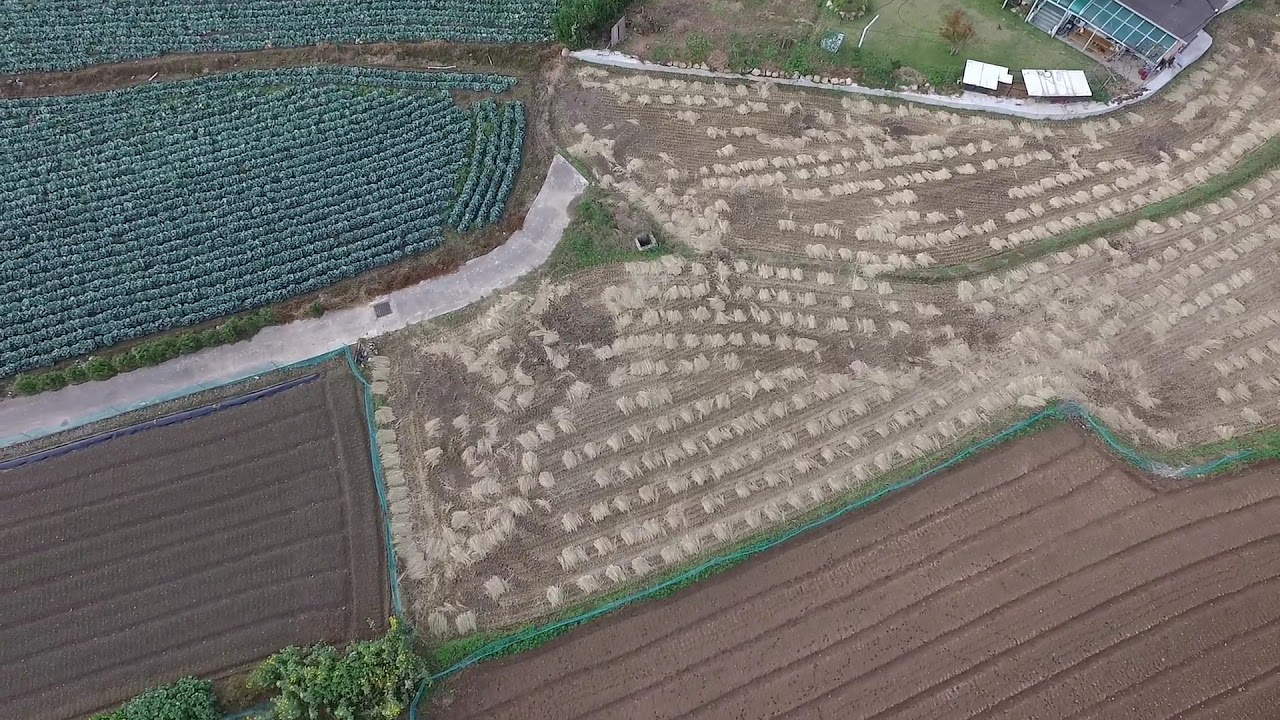This aerial view of farmland captures a diverse agricultural landscape divided into distinct sections. In the lower left-hand corner, we see a field with dark brown rows of freshly tilled soil, awaiting planting. Adjacent to it, in the lower right-hand corner, another field shows diagonal rows of bare dirt, similarly prepped for sowing. Between these two fields, a cluster of green trees adds a touch of natural greenery. Above them, neatly aligned rows of baled hay stretch across the central part of the image. In the upper left-hand quadrant, a vibrant bluish-green crop thrives in neatly planted rows, its lushness contrasting with the dry, yellowed grass spotted near the center and right. Further up, in the upper right-hand corner, a farmhouse with a well-maintained yard is situated, featuring patches of green grass and brown dirt. Nearby, a greenhouse with a glass roof and two aluminum-roofed sheds underline the functional aspects of the farm. A road can be seen dividing the healthy green crop area from the drier, less fertile sections of the land, graphically illustrating the varied uses of the farmland.